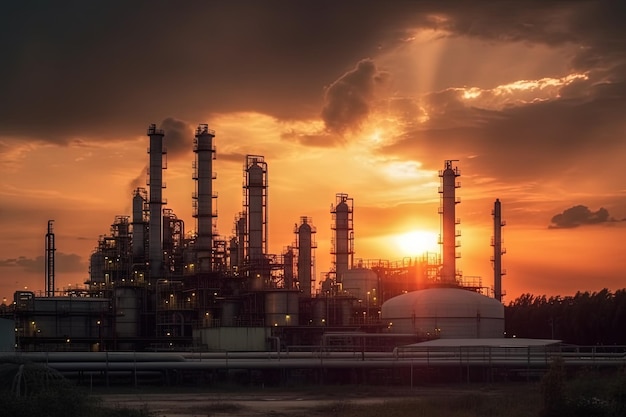In this distant, high-quality photograph of an oil refinery captured at sunset, the scene is dominated by the tall, intricate towers and spires of the industrial plant, silhouetted against a sky painted in hues of orange and yellow. The sun, partially obscured by clouds, casts a warm glow over the facility, while beams of light pierce through, illuminating the complex network of structures including smokestack-like refining cylinders and scaffolding. In the foreground, large white containment tanks stand prominently, with dark, brownish waters stretching out in front. The entire refinery is adorned with shimmering lights, creating a striking contrast against the dusk sky. To the right, a tree line frames the industrial scene, adding a natural boundary to the engineered landscape.